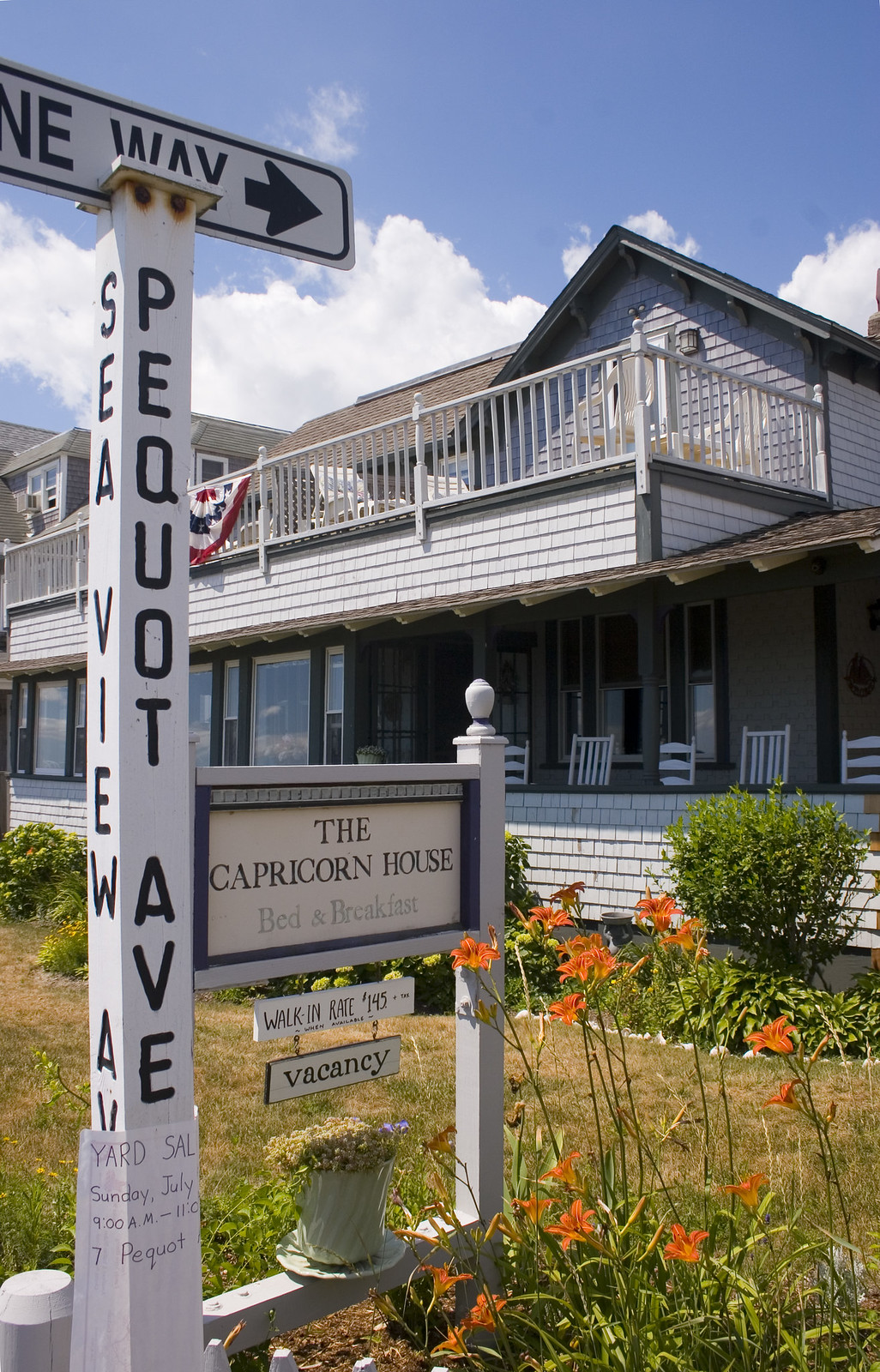This detailed caption synthesizes the provided information:

The photo captures the exterior of "The Capricorn House Bed-and-Breakfast," a charming two-story country cottage-style residence with light gray or white siding. The house has black-framed windows and a wraparound porch adorned with multiple white rocking chairs. A notable feature is the open-air deck on the second floor, furnished with lawn or plastic lounge chairs. In front of the bed-and-breakfast, there is a well-manicured garden brimming with vibrant flowers, prominently featuring orange lilies.

A significant element in the foreground is a white wooden signpost. The rectangular sign hanging from it reads "The Capricorn House Bed-and-Breakfast" in black text, advertising walk-in rates at $145 plus tax and displaying a vacancy sign beneath it. Adjacent to this signpost, additional signage includes a "One Way" sign at the top with an arrow pointing to the right, and directional signs for "Pequot Avenue" and "Seaview Avenue." A smaller piece of paper attached to the post advertises a yard sale. The scene evokes a serene, welcoming atmosphere typical of a picturesque country retreat.